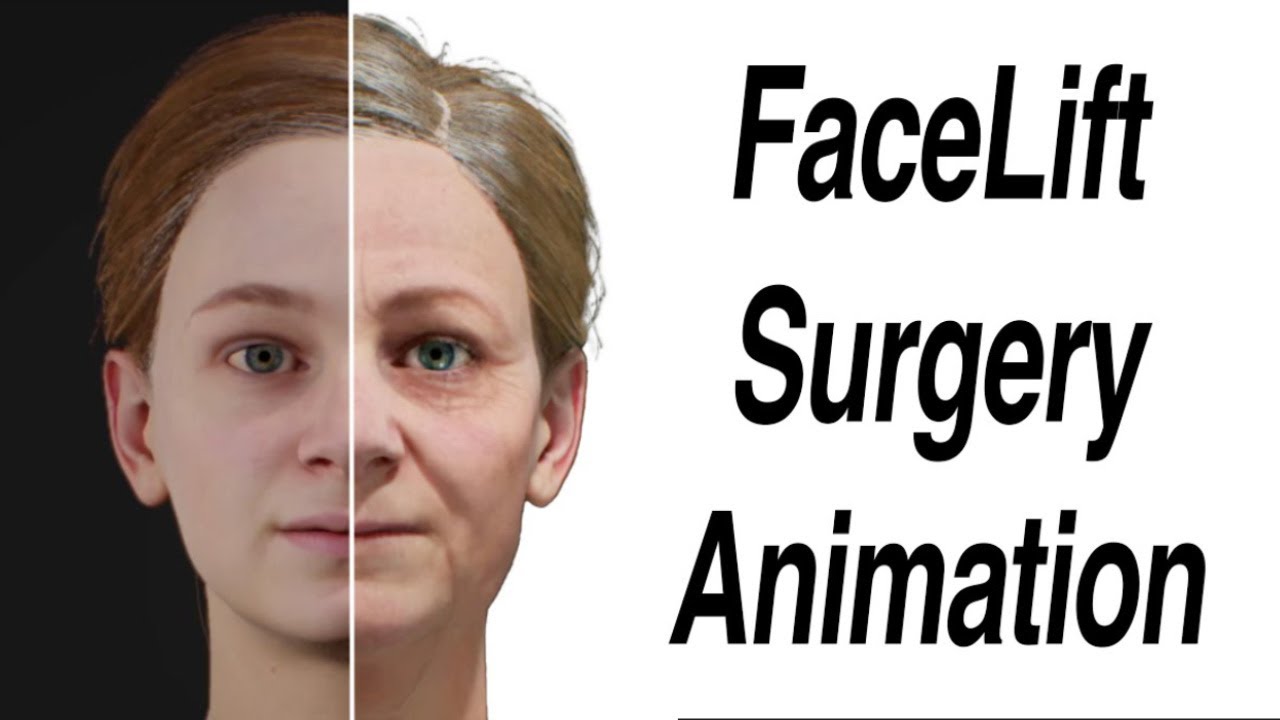The image is a promotional ad for facelift surgery animation. It features a digitalized depiction of a person, possibly a woman or man, with half of the face against a black background and the other half against a white background. The right side of the image prominently displays the words "facelift surgery animation" in bold black text.

The face itself is divided to illustrate a dramatic before-and-after effect of a facelift procedure. The left side of the face, set against a black background from the viewer's perspective, appears considerably younger with vibrant, possibly dyed hair and virtually no wrinkles, resembling a 20-year-old. In contrast, the right side of the face, set against a white background, looks much older with gray hair and numerous wrinkles around the eyes, forehead, nose, and mouth, suggesting the appearance of a 50-year-old. The neck on the older side also appears somewhat droopy. 

The image employs stark contrasts and lighting to effectively highlight the potential transformative effects of facelift surgery, presenting a sharp visual dichotomy between youthful rejuvenation and aging.